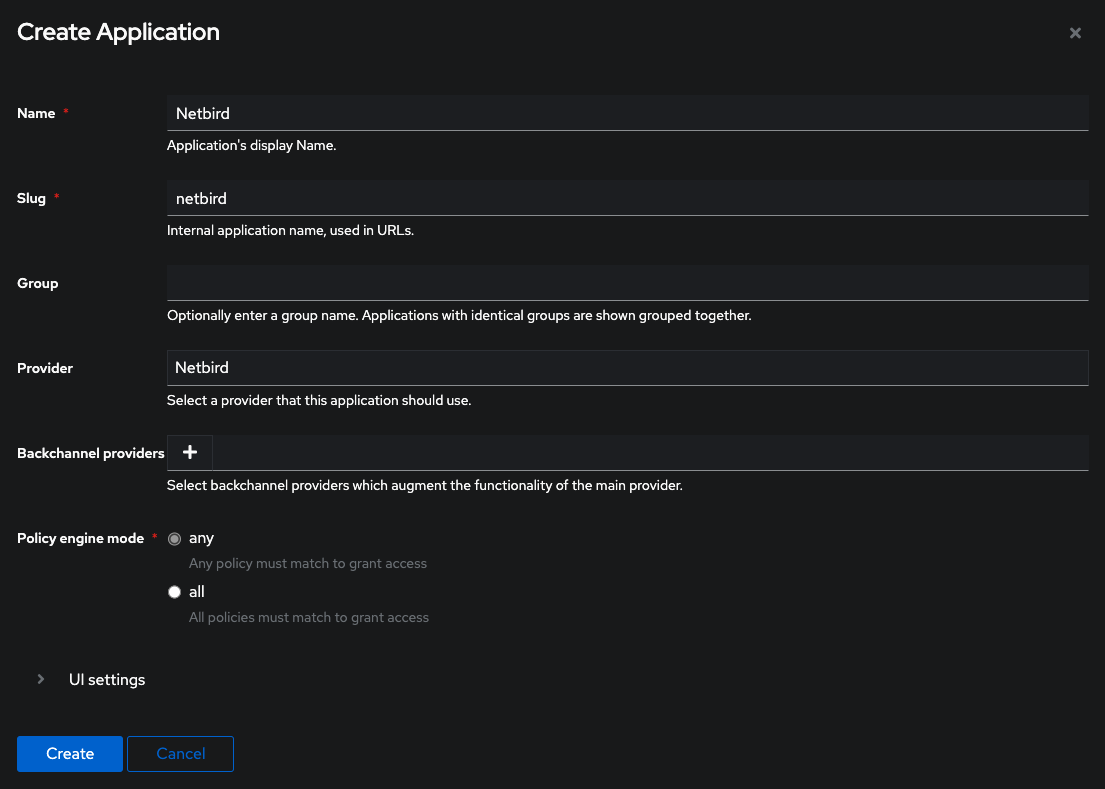The image showcases a sign-up form within a web or mobile application, designed for creating a new application on the platform. The form has a sleek black background and contains several input fields and interactive elements.

At the top of the form, the heading reads "Create Application." Below the heading, there are five primary text fields, each accompanied by a brief description:

1. **Name**: This field is intended for the display name of the application. In this example, the user has entered "Netbird."
2. **Slug**: Defined as an internal application name used in URLs, the same name "Netbird" has been inputted here.
3. **Group**: This optional field allows users to enter a group name to categorize applications with identical group names together. The field is currently empty in the image.
4. **Provider**: The user entered "Netbird" in this field, which specifies the provider the application should use.
5. **Backchannel Providers**: Accompanied by a plus icon, this field instructs users to select backchannel providers that will augment the main provider's functionality. This field also appears to be empty.

Below the text fields, there are radio buttons to configure the "Policy Engine Mode". The two options available are:
- "Any policy must match to grant access"
- "All policies must match to grant access"

Further down, there is a collapsible menu labeled "UI Settings", hinting at additional configuration options for the application's user interface. At the bottom of the form, two prominent buttons provide the options to "Create" or "Cancel" the new application setup.